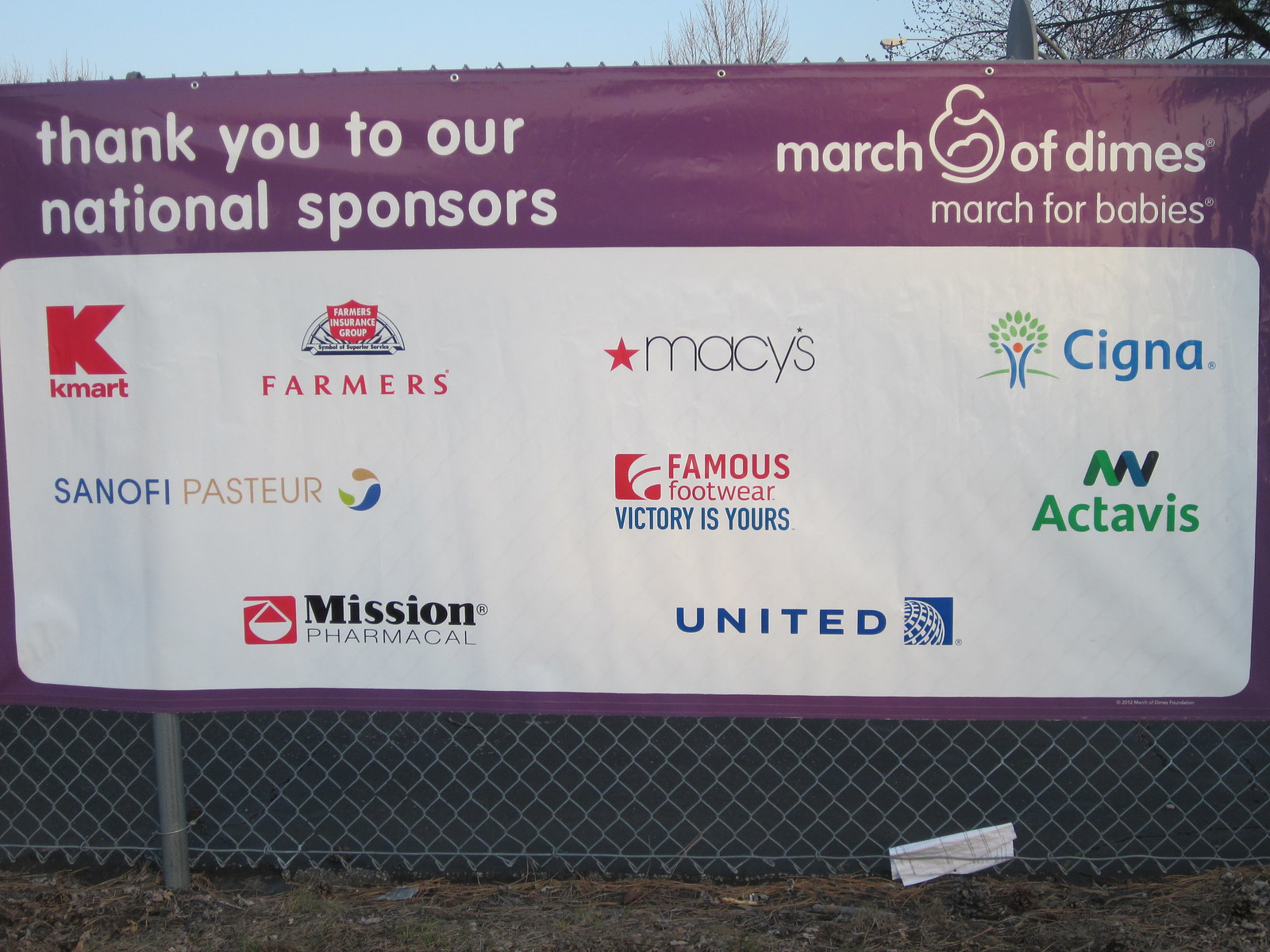This photograph captures a vibrant outdoor scene featuring a detailed banner mounted on a metallic chain link fence. The banner, which has a purple border and a white central panel, prominently displays a heartfelt message in white lettering: "Thank you to our national sponsors." This is accompanied by logos and mentions of March of Dimes and the March for Babies initiative. Below this message, set against the white background, are logos of several sponsors, including Kmart, Farmers, Macy's, Cigna, Sanofi, Famous Footwear, Actavis, Mission Pharma, and United. The banner is attached to the interior side of the fence, which stands in front of some dirt grounds, devoid of grass. Behind the fence, the scene extends to reveal a clear blue sky framed by branches from nearby trees and a dark grey tarp partially covering the fence. Additionally, there's a piece of paper affixed at the bottom of the fence, adding a subtle detail to the vibrant outdoor setting.